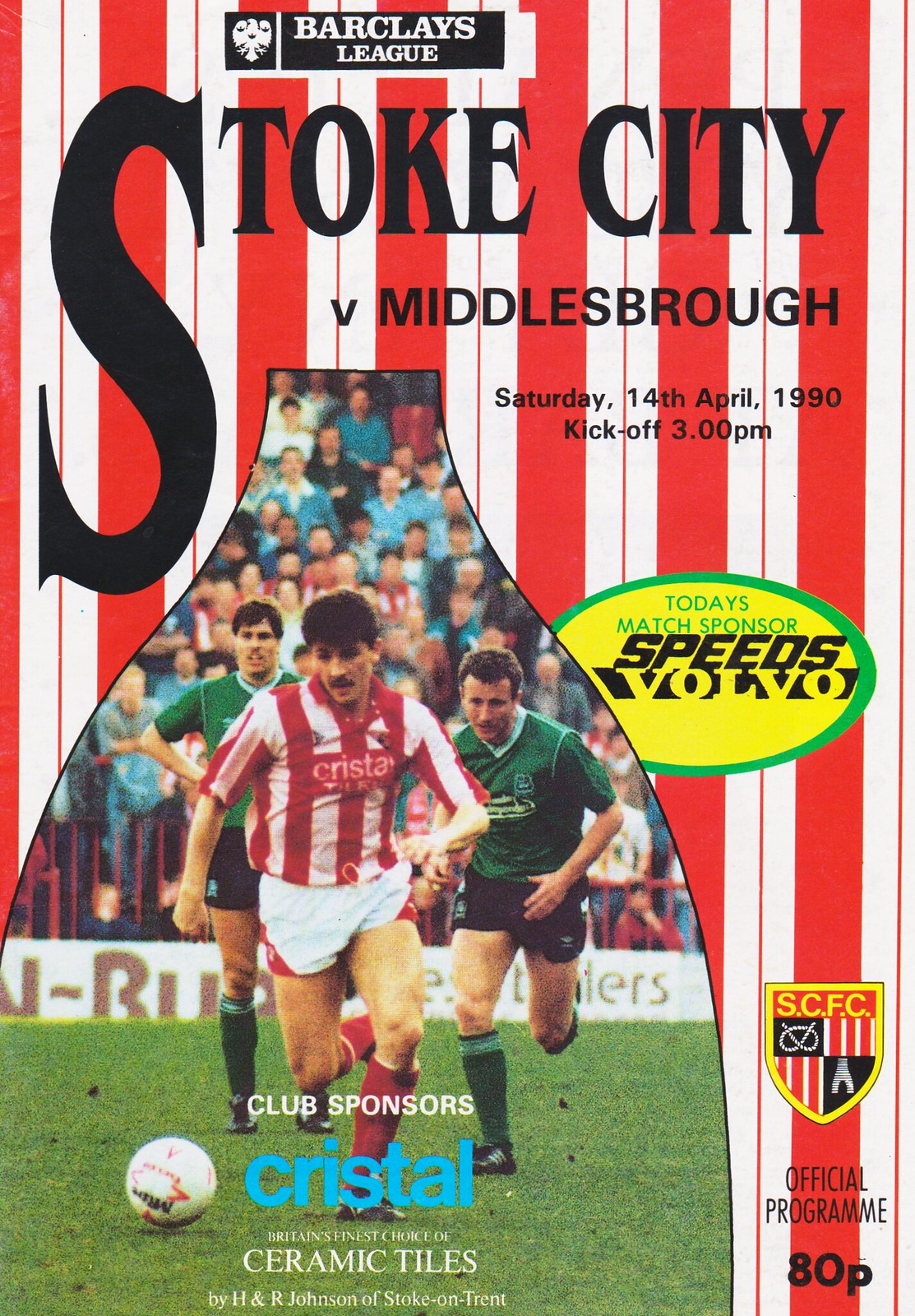The image depicts the official program cover for a Barclays League soccer match, dated Saturday, 14th April, 1990, with kickoff at 3 p.m. The program features a prominent large "S" in black font at the top, spelling out "Stoke City" versus "Middlesbrough" below in smaller black font. The backdrop consists of red and white vertical stripes, mirroring the uniform of one of the central players. At the top left, there is a bird crest to the left of the Barclays League emblem, which is displayed in white font on a black rectangular background.

In the center of the cover is a photograph shaped like a bottle, showcasing three soccer players: one in a red and white striped jersey with "Crystal" as the sponsor, controlling the ball, and two players in green uniforms, with one actively pursuing the player with the ball and another standing in the background. The player in the red and white jersey is also wearing white shorts with red stripes and red socks, while the players in green have black shorts. 

Around the bottle-shaped image, various pieces of text highlight that Speeds Volvo is the match sponsor and Crystal is the club sponsor, with additional sponsorship noted from H&R Johnson of Stoke-on-Trent for ceramic tiles. The program, labeled as the official match program, has a price marked at 80p. 

Overall, the cover combines essential match details, sponsorships, and a vivid action shot of the players, superimposed on a background that matches the team's uniform theme for added visual continuity.